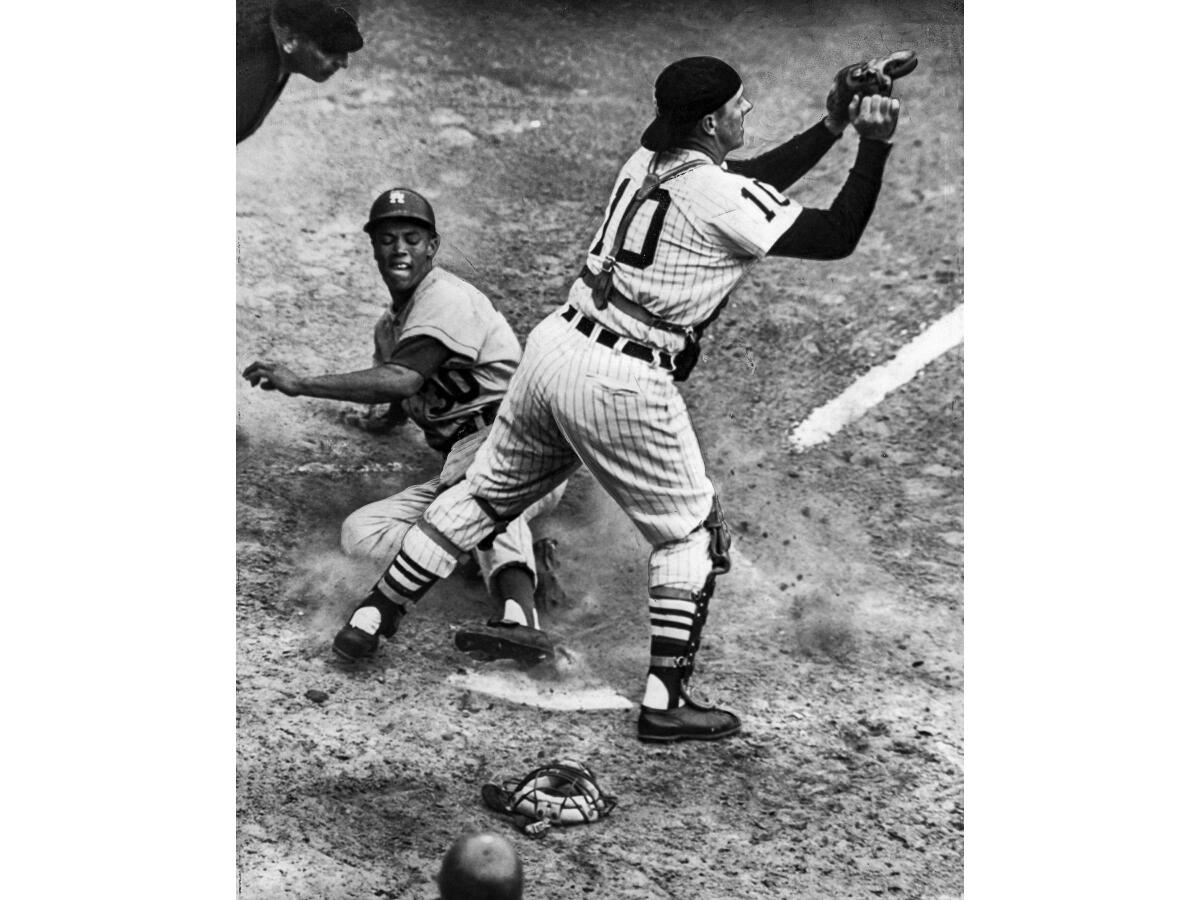This black-and-white photograph captures a dramatic moment from an old baseball game, characterized by its gritty texture and historical ambiance. It depicts a player from the away team, wearing an LA Dodgers helmet and the number 30 jersey, sliding into home base with intense determination. The player’s foot is seen sliding directly between the legs of the catcher, who is adorned in number 10 with black knee guards, a black hat worn backward, and black sleeves under his jersey. The catcher, seemingly from the Yankees, stands poised to catch a ball that is not yet in the frame, with his mask discarded on the ground nearby. The umpire, dressed in all black, is stationed in the top left corner, carefully observing to determine if the player is safe. An additional player, wearing a helmet, watches intently from the background. This photograph, likely from the 1960s given the attire and equipment, conveys the suspense and athleticism of a slide into home base, capturing a snapshot of baseball history in vivid detail.